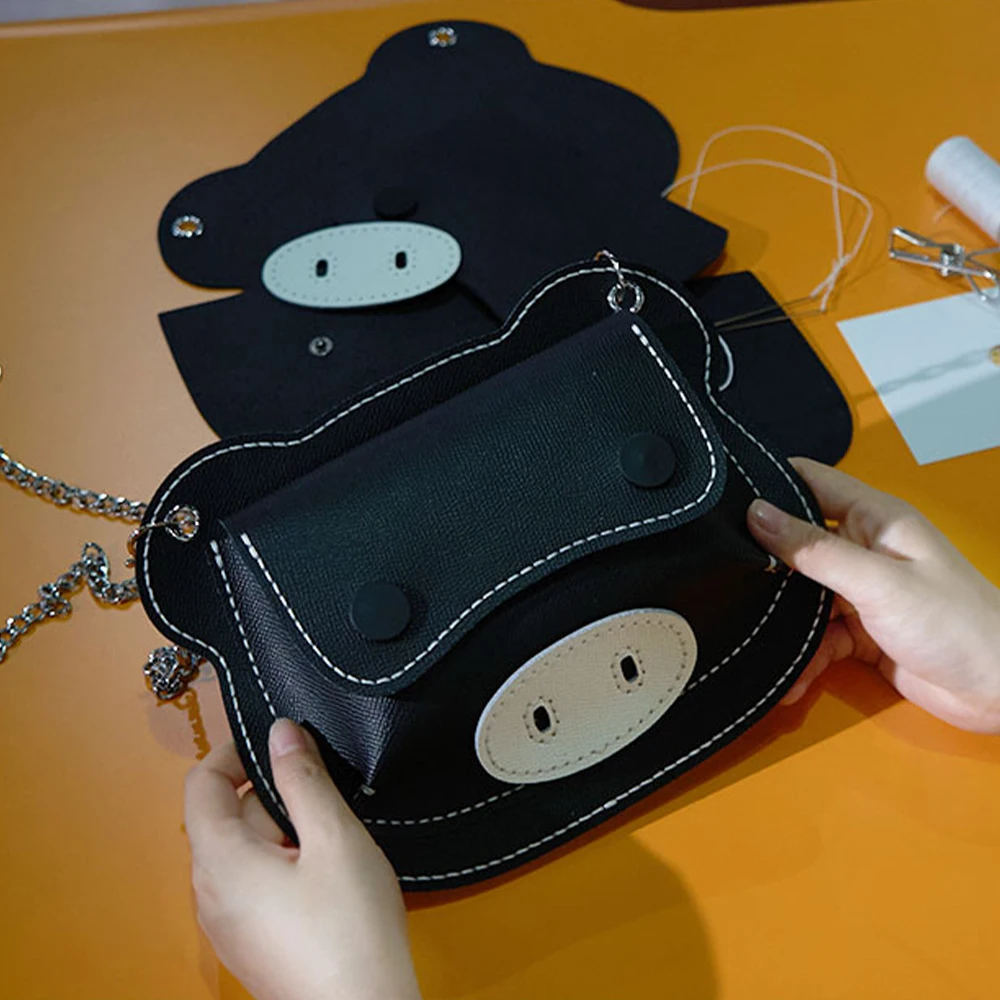This photograph features a detailed close-up of a handcrafted purse shaped like a whimsical, cartoonish pig's head. The black purse, which is accentuated with white stitching, has two black buttons resembling eyes and a white oval snout with stitched details and two holes mimicking nostrils. A metal chain, passing through silver holes positioned where the pig's ears would be, serves as the purse strap. The setting includes two hands prominently displaying the finished product against a bright, smooth orange background.

On the surface around the purse, various materials and tools used in its creation are visible. These include black pieces of fabric and additional white leather-like material similar to the snout. You can also spot a spool of white yarn, sewing needles threaded with the same yarn, and a pair of silver scissors. The golden-orange-yellow table upon which these items are arranged adds a vibrant contrast to the overall scene, further highlighting the meticulous crafting process.